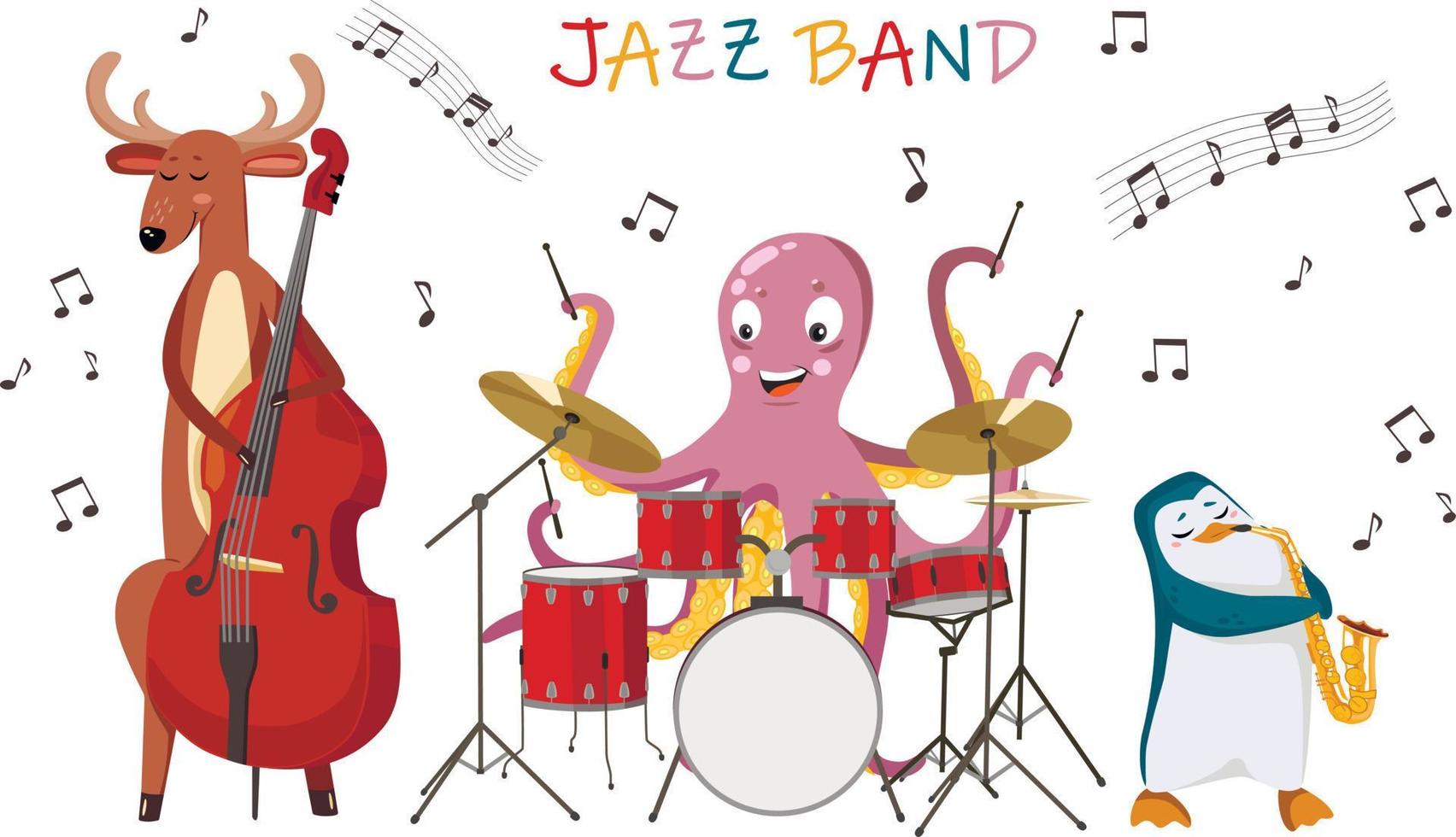The detailed cartoon illustration portrays a vibrant jazz band consisting of three cheerful animals passionately playing their instruments against a crisp white background. At the center is a pink octopus, enthusiastically playing a set of red drums with drumsticks in four of its tentacles. On one side, a brown reindeer, eyes closed in concentration, expertly plays a matching red cello with musical notes floating upwards. On the other side, a blue and white penguin, deeply engrossed in the music, plays a saxophone, emanating more musical notes. Above them, the phrase "Jazz Band" is spelled out in colorful, individual letters, adding to the whimsy of the scene. The entire image exudes a lively and colorful atmosphere, with musical notes scattered throughout, illustrating the joyful harmony of the performance.